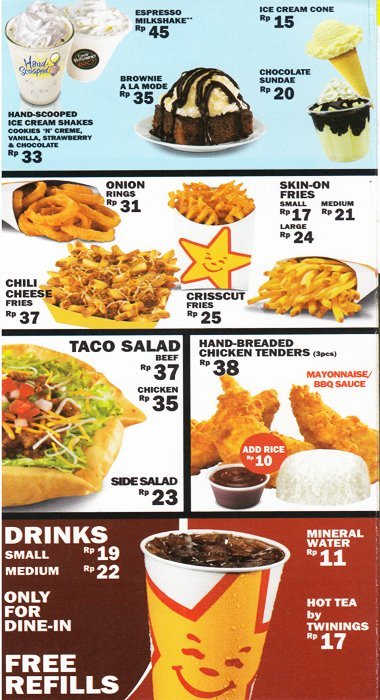This is a detailed advertisement menu from a fast food restaurant, likely Carl's Jr. or Urby's, recognized by the prominent star logo with a smiling face in the center. The menu is divided into sections starting from the top showcasing a variety of desserts. The top section features hand-scooped ice cream shakes in flavors like cookies and cream, vanilla, strawberry, and chocolate, alongside a brownie a la mode and a chocolate sundae served in a clear cup. An ice cream cone is also listed, prominently priced at RP15.

Below the desserts, the menu highlights side orders, including onion rings labeled RP31 and various sizes of "skin-on" fries in small, medium, and large, with prices 17, 21, and 24 respectively. Also featured are chili cheese fries in a yellow container priced at RP37, regular fries, and crisp cut fries at RP25.

The next section introduces the taco salad available with chicken, beef, or as a side salad, alongside hand-breaded chicken tenders priced at RP38. A red circle with the note "at price 10" accompanies a container of red sauce labeled mayonnaise and barbecued chicken.

At the very bottom, the drink selection is shown, where din-in only options come with free refills. Sizes are priced, with small at 19 and medium at 22. The central graphic displays a soda cup featuring the star logo with a red smiley face. On the right side, listings include mineral water for 11 and Twin's hot tea at RP17.